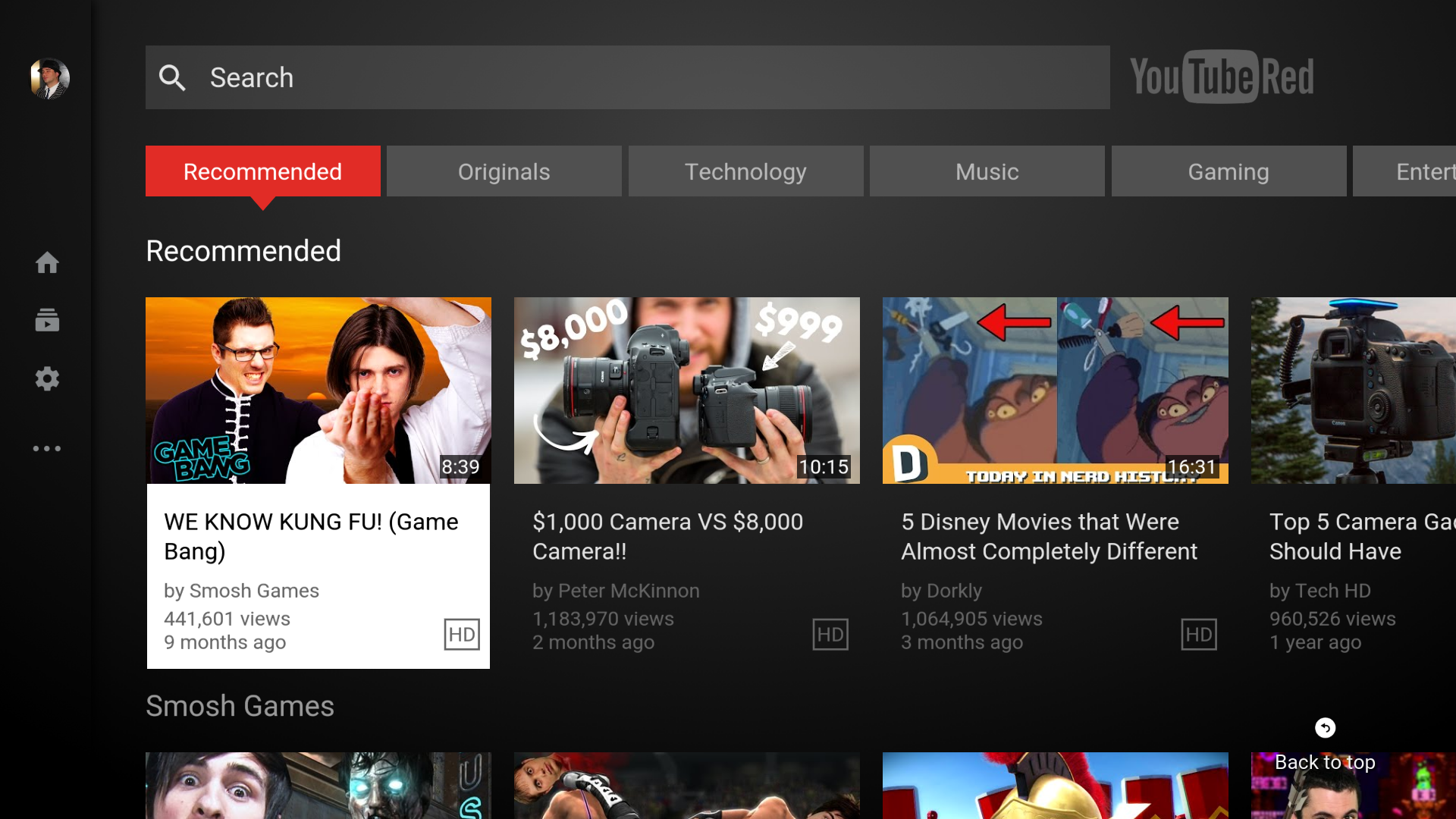The image resembles a desktop wallpaper and prominently features the interface of a video streaming platform, likely YouTube. The overall backdrop is black, creating a stark contrast with various interface elements. On the left side of the screen, there is a vertical sidebar. At the top of this sidebar, there is a circular thumbnail depicting a man in a gray suit and white shirt. Below the thumbnail, aligned vertically, are icons indicative of different functions: a house icon, a play button, a gear, and three dots. 

Positioned at the top of the screen is a gray search bar. To its right, the YouTube logo is displayed in red and gray colors. Below the navigation bar is a horizontal menu featuring categorically organized bars: 'Recommended' (highlighted in red), 'Originals,' 'Technology,' 'Music,' 'Gaming,' and 'Entertainment.'

Under the 'Recommended' section, a horizontal list showcases four rectangular thumbnail images, each representing a different video. 

1. The first thumbnail depicts two males; one wears a white shirt, and the other wears a black shirt with a white center stripe. The video title reads, "We Know Kung Fu, Game Bang by Smosh Games," accompanied by the text "441,601 views, nine months ago."
2. The second thumbnail shows a person holding two cameras, labeled "$1,000 Camera vs. $8,000 Camera."
3. The third thumbnail features an animated character with a red arrow at the top. Its title reads, "Five Disney Movies That Were Almost Completely Different."
4. The fourth thumbnail displays an image of a camera with the partial text "Top Five Cameras..." and "GA... should have."

The detailed interface layout and the engaging video suggestions make this desktop wallpaper both informative and visually appealing.